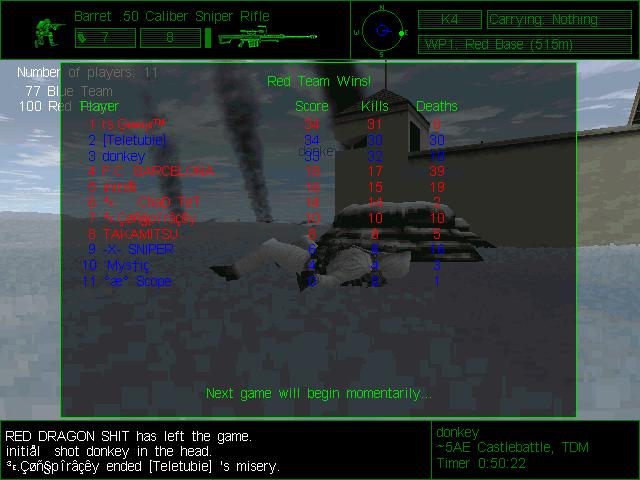The image is a detailed screenshot from the end screen of a shooter video game. Dominating the top of the screen is the announcement "Red Team Wins," written in bold. A digital box in the center contains detailed statistics of the game, showcasing the players' names, scores, kill counts, and deaths. The box has a thin green border and a grayed-out interior, with the rest of the vivid game scene visible in the background.

The screen features various colored texts: red, blue, green, and white. A green text at the bottom reads "Next game will begin momentarily." An interface showing game-related data, such as "Barrett 50 Caliber Sniper Rifle" and a soldier holding a rifle, is prominently displayed in the top left corner. Other elements include the numbers 7 and 8, and additional labels like "K4 carrying nothing," "WPA1," and "Red Base, 515 meters."

Behind the statistics box, the game's environment is slightly visible. There's a blue sky with scattered clouds and some gray smoke emanating from three different areas in the background. A character, dressed in gray and appearing to have been shot, lies on the dark gray ground. At the bottom, white text provides a chat log with messages such as "Red Dragon Shit has left the game," "Nisha was shot," and other descriptions that seem to recount game events, adding to the immersive post-game detail.